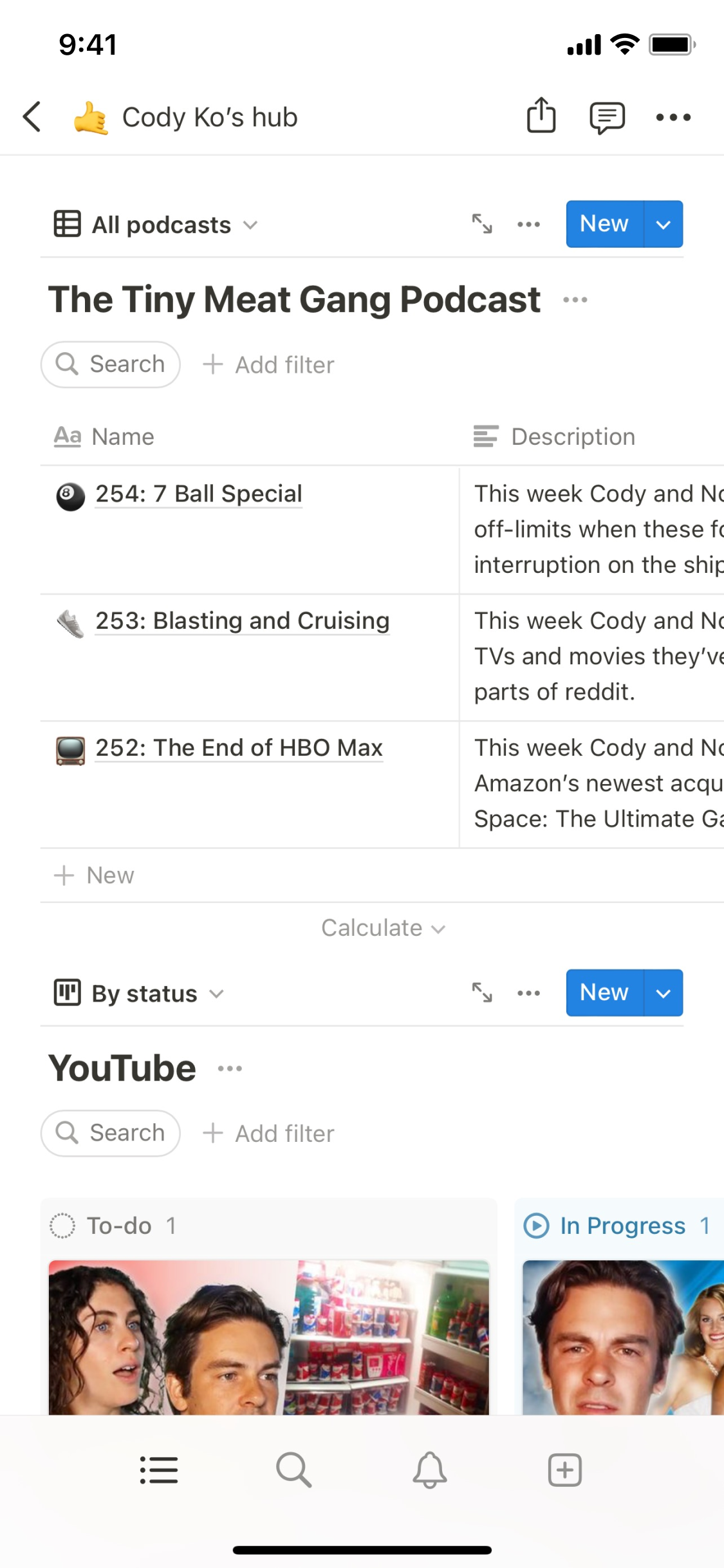The image appears to be a screenshot taken from a smartphone, depicting content related to a YouTube video, likely featuring a podcast. At the top, the screen displays the current time, 9:41, alongside indicators for Wi-Fi connection strength and battery level. Beneath these indicators, there is a search bar labeled "Cody's Co-Hub," accompanied by a sharing symbol, represented as a square with an arrow pointing out of it.

Dominating the screenshot is a post highlighting the "Tiny Meat Gang Podcast." It contains detailed descriptions of the podcast, including names of the hosts and the topics covered. A list resembling a calendar and additional narrative descriptions are also visible.

Towards the bottom of the screenshot, options to sort the content via different filters are presented. Additionally, there are thumbnails of related YouTube videos featuring various individuals. The bottom toolbar includes several icons, such as a magnifying glass for search functionality, an alert button for notifications, and a square with a plus sign, potentially for adding new content or bookmarks.